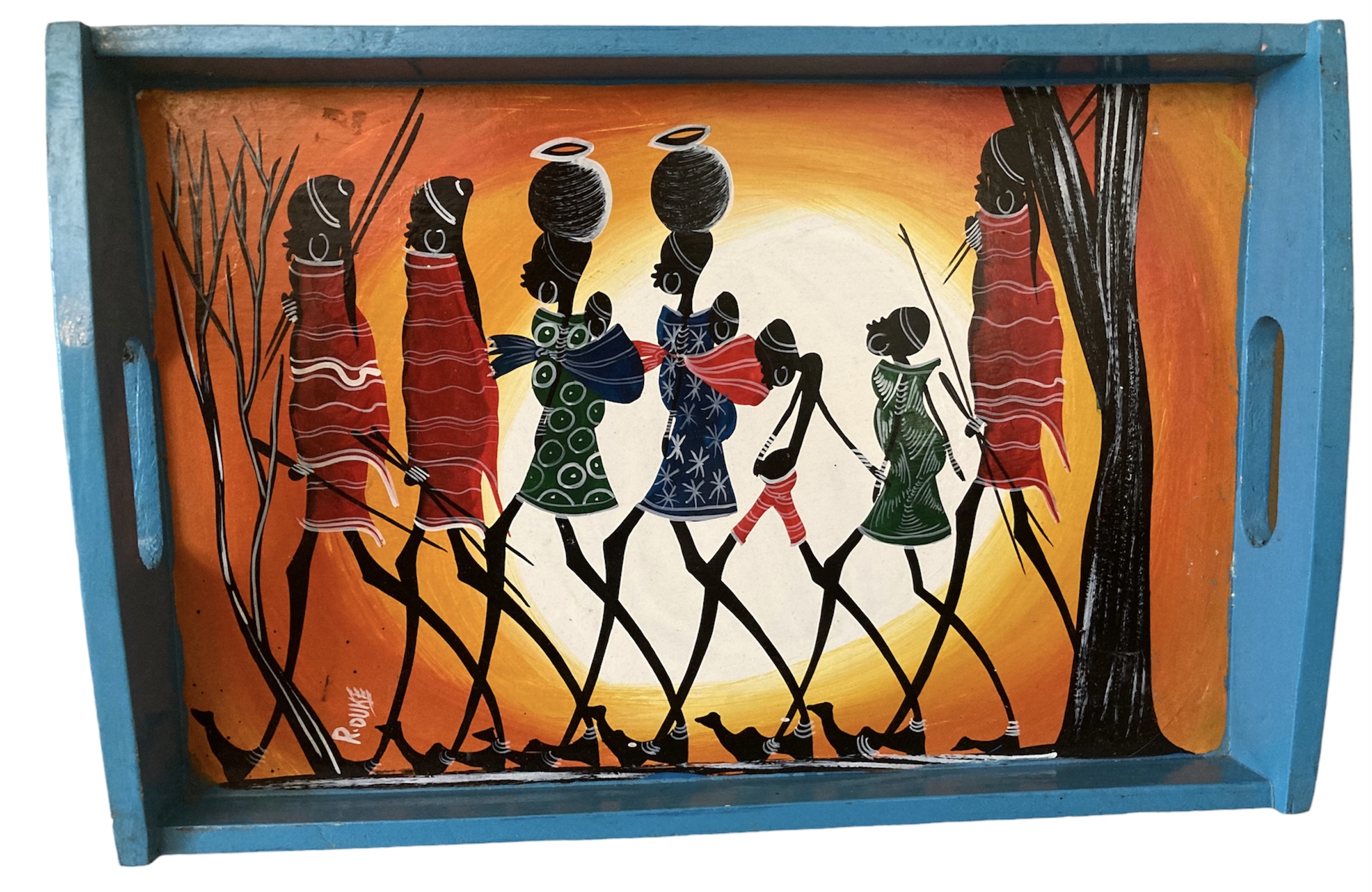The image is framed by what looks like a blue TV tray with handle-like protrusions in the middle of both the left and right borders, giving it a sense of depth. Inside this frame is a vibrant painting, likely depicting an African scene. The background is predominantly orange, with a large sun occupying much of the mid-section, radiating yellow hues that blend into the orange, extending to the edges of the painting. 

At the forefront, there are seven figures walking from right to left, resembling stick figures but adorned in colorful attire that appears culturally significant. These characters, presumed to be African women, are dressed in a variety of vividly patterned outfits. The two leading figures on the left are clothed in red blankets adorned with horizontal white stripes, and they wear dark caps with white stripes at the bottom. Each has an earring in their left ear. 

Behind them, a woman with a distinctive headdress features a large grayish ball with an orange center and white rim, and she wears a green dress topped with an oversized blue bow. Directly following her is another woman in a similar headdress, but with a blue dress patterned with white stars and a large pink bow.

Continuing towards the right, the next two characters are slightly shorter; one is partially hidden, showing only a bent-over head and a pink garment that reaches just above the knee. The other looks upwards and sports a green outfit with white accents.

The final and tallest figure, dressed similarly to the front two in a red robe with white stripes, holds something under her right arm that extends behind her head and behind a thick tree at the right edge of the painting.

The scene also features natural elements, including a thin, branchy tree without leaves towards the left, and a thicker tree trunk on the right, which splits into two branches extending out of the image. The overall composition, with its bold colors and cultural hints, creates an evocative mosaic of life likely set at sunset, adding an ethereal glow to the scene.